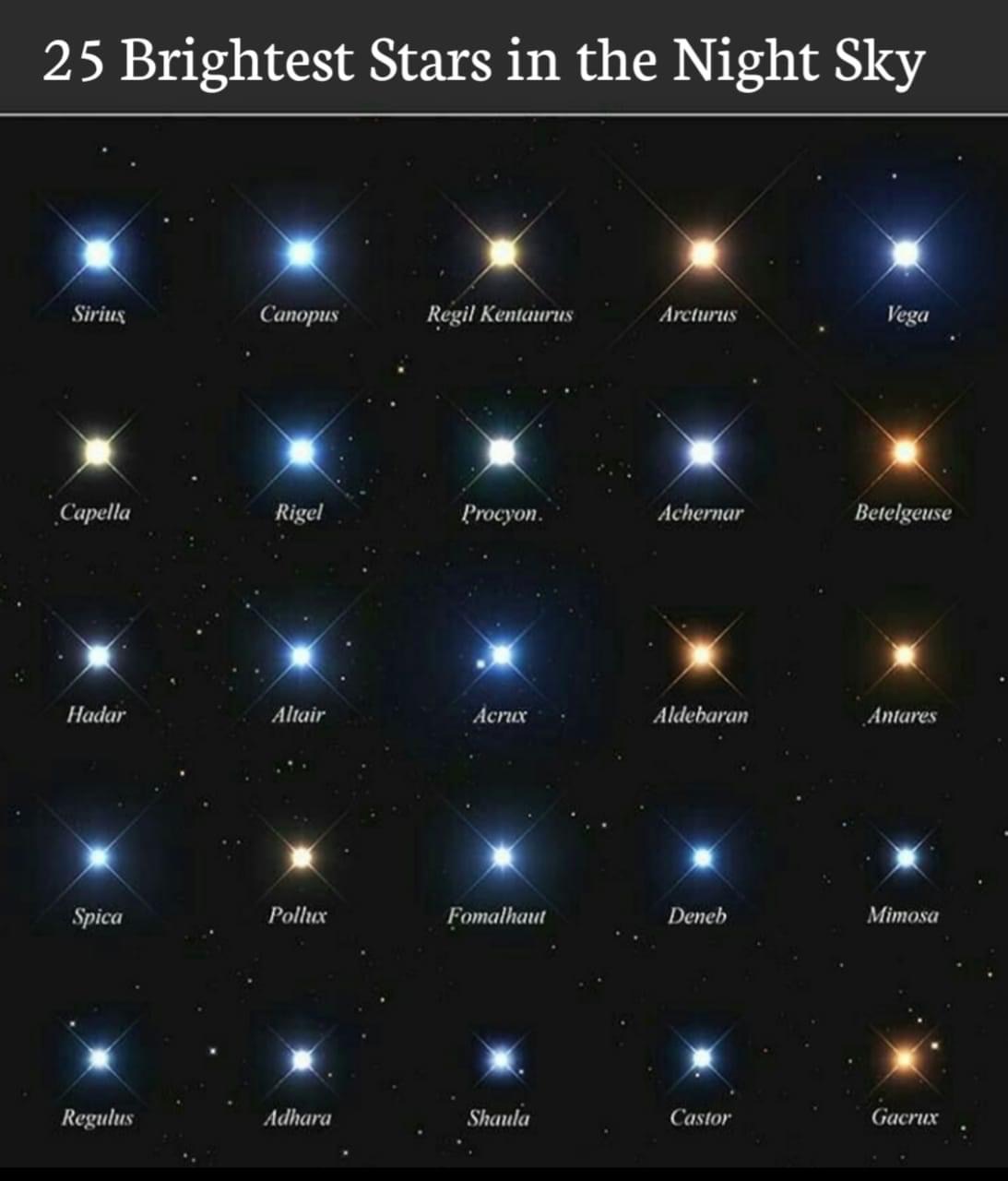The poster titled "25 Brightest Stars in the Night Sky" prominently displays this title in white text against a solid black background, underlined by a horizontal white line at the top. The layout features five rows of stars, each containing five stars, totaling the 25 brightest stars. Each star is depicted in its natural color, with common hues being white, blue, and yellow. The background simulates space, dotted with smaller stars. Starting from the top left, the first star is Sirius, which is white. Other notable stars include Arcturus (yellow), Canopus, Rigel, and Vega. The array showcases the varying brightness and color tints of each star against a backdrop of the night sky, emphasizing their prominence in the celestial panorama.